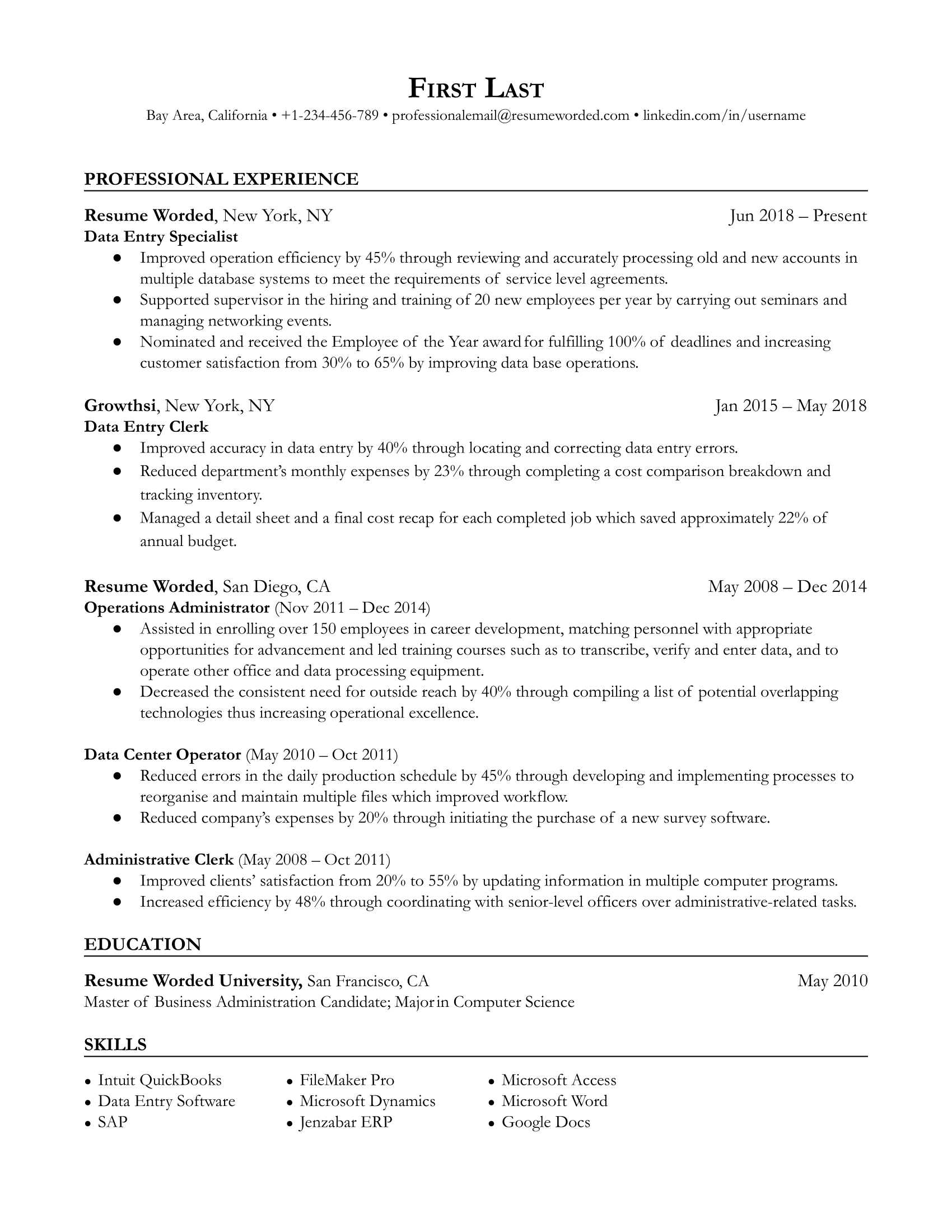This image showcases a detailed, professionally typed resume in black text. At the top, it features the placeholder name "First Last," followed by the location "Bay Area, California," a phone number "123456789," a professional email address "resumeworld.com," and a LinkedIn URL "linkedin.com/in/username."

The resume is divided into several sections with headers including "Professional Experience," "Education," and "Skills," each marked by black underlined dividers. The "Professional Experience" section highlights roles such as Data Entry Specialist at "Resume Awarded" in New York, New York, from June 2018 to present, with associated bullet points detailing responsibilities. Other positions listed include Data Entry Clerk at "Grousey" in New York, New York (January 2015 to May 2018), Operations Administrator at "Resume Awarded" in San Diego, California (May 2008 to December 2014), Data Center Operator (November 2011 to October 2011), and Administrative Clerk (May 2008 to October 2011), each with bullet points describing job duties.

In the "Education" section, it notes "Resume Awarded University" in San Francisco, California, with a Master's of Business Administration Candidate majoring in Computer Science, attained in May 2010.

The "Skills" section itemizes proficiency with various software and tools including Intuit QuickBooks, SAP, FileMaker Pro, Microsoft Dynamics, JezBar, ERP, Microsoft Access, Microsoft Word, and Google Docs.

This comprehensive resume clearly outlines the candidate's professional journey, educational background, and technical expertise.